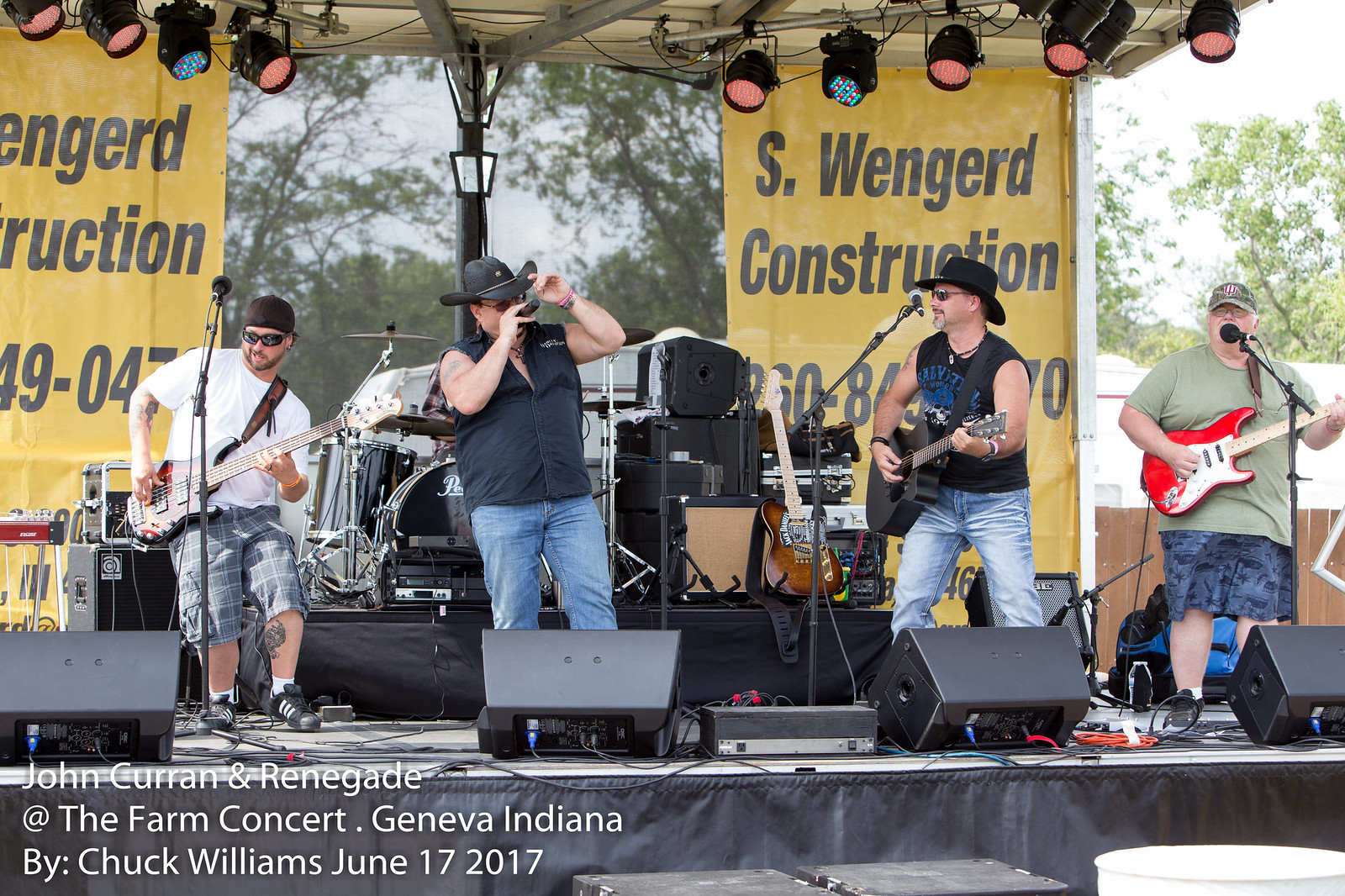In this detailed outdoor photograph taken during the daytime, a stage setup is seen with a backdrop of trees, branches, and a bluish-gray sky. The banner on the stage reads "John Curran and Renegade at the Farm Concert, Geneva, Indiana," credited to photographer Chuck Williams on June 17th, 2017. On the stage, marked by a black curtain at the bottom and illuminated with rows of spotlights overhead, there are five musicians performing.

From left to right, starting with a guitarist in a white T-shirt and gray shorts, the image progresses to show a drum set partially hidden behind the musicians. The next performer wears a backward hat with sunglasses and plays either a guitar or bass. Beside him is a burly man in a black sleeveless shirt and blue jeans, wearing a black cowboy hat and holding a microphone, indicating he is the lead singer. Another individual, wearing a black tank top and cowboy hat, also plays an acoustic guitar close to him. On the far right stands a slightly older man in a light green short-sleeved T-shirt with blue shorts, holding a red guitar.

In front of the performance area sit four black speakers, supplying sound for the event. The backdrop includes yellow banners from S. Wengard Construction, partially cut off but replicated on both sides of the stage. The overall setup and attire of the performers create an authentic, casual concert atmosphere.